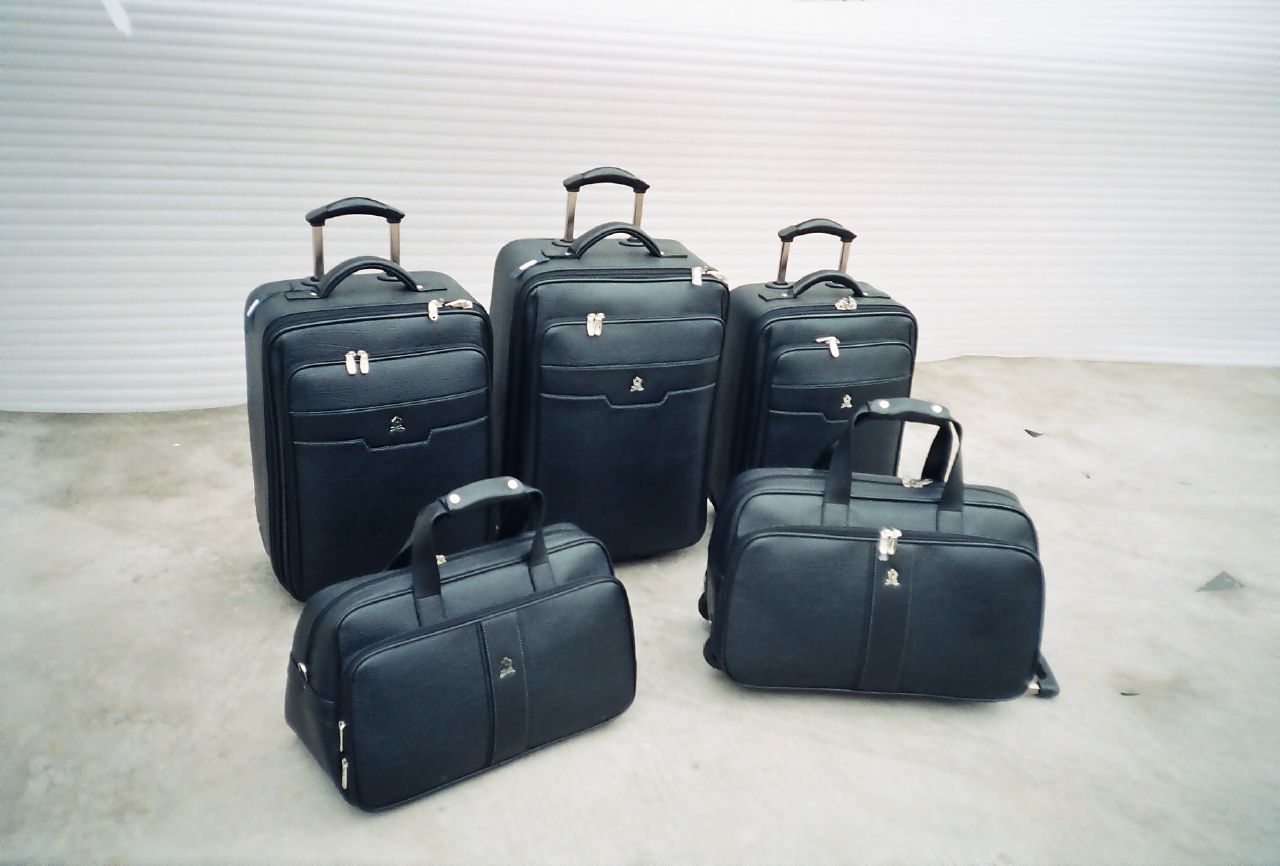The image displays a meticulously arranged luggage set, likely intended for a product advertisement. The backdrop is a textured white wall taking up about a fourth of the frame, with horizontal lines running across it and a bright flash reflecting off the upper center to right portion. The remaining space is dominated by a gray concrete floor. The main focus of the photo centers on five stylish black leather suitcases, each adorned with gold-colored zippers and accents, topped with silver metal bars and black handles. 

In the back row, three rolling suitcases are lined up, with the extendable handles partially pulled out. The center suitcase is the largest, flanked by slightly smaller ones on either side. In front of these, two black leather duffel bags are positioned at an angle, their handles neatly brought together. The duffel bags also sport a gold logo in the center, complementing the overall luxurious appearance. The composition and high-quality lighting suggest that this photo is crafted to showcase the premium nature of the luggage, making it suitable for use in online advertisements or e-commerce sites.